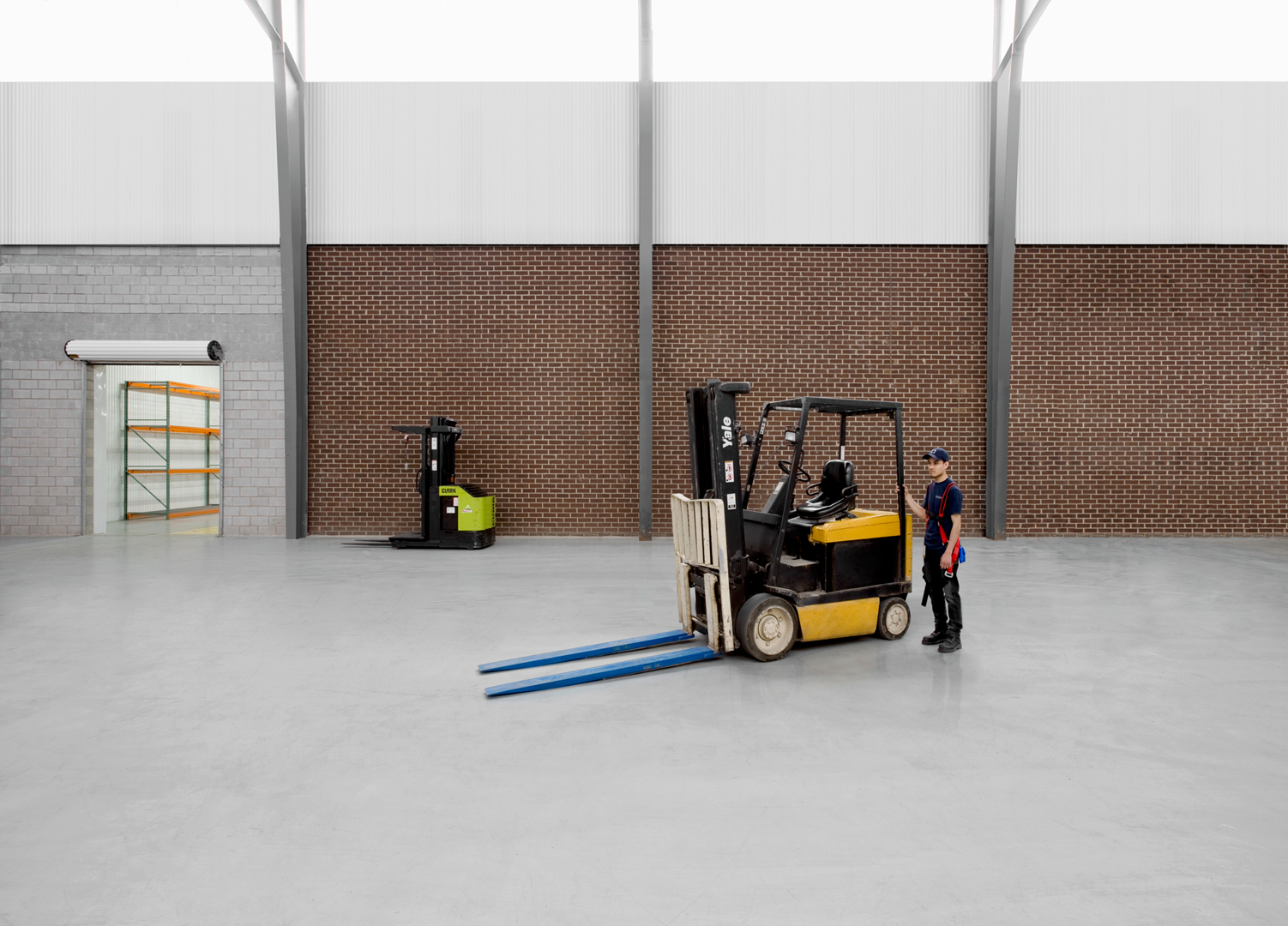The image depicts a spacious, clean warehouse with concrete floors and a mix of red brick and white brick walls. Central to the photograph is a black and yellow forklift with blue tongs, positioned slightly to the center-right. A man, wearing a blue and black uniform along with a blue baseball cap, stands next to the forklift, holding its back and looking into the distance. To the back left of this forklift, there is a smaller green and black stand-up forklift. The color palette of the image includes grays, reds, whites, yellows, greens, blues, and blacks. On the left side of the warehouse is an open doorway leading to another room with an empty shelf visible through the opening. The setting suggests a large, mostly empty industrial space dominated by the forklifts and the man inspecting them.